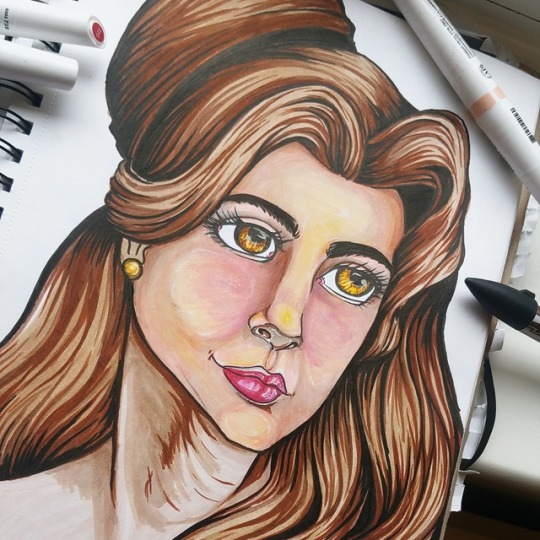In this photograph of a drawing, a white sketch pad with a black spiral binding dominates the image, almost filling the entire frame. The sketch pad rests on an unidentified surface, and a few markers lie on top of it, suggesting they were used in the creation of the artwork. 

The drawing itself features a highly detailed and realistic portrait of a woman. She appears to be of Caucasian descent and has long brown hair accentuated with various highlights in off-white and pale yellow tones. Her face is intricately rendered, showcasing heavy makeup that includes dark eyebrows, large amber-brown eyes adorned with prominent eyelashes, and strikingly red lips. One of her ears is visible, adorned with a small gold stud earring. The texture of her neck is meticulously detailed, adding to the lifelike quality of the sketch. The woman's long hair extends beyond her shoulders, contributing to the overall sense of realism in this impressive piece of art.